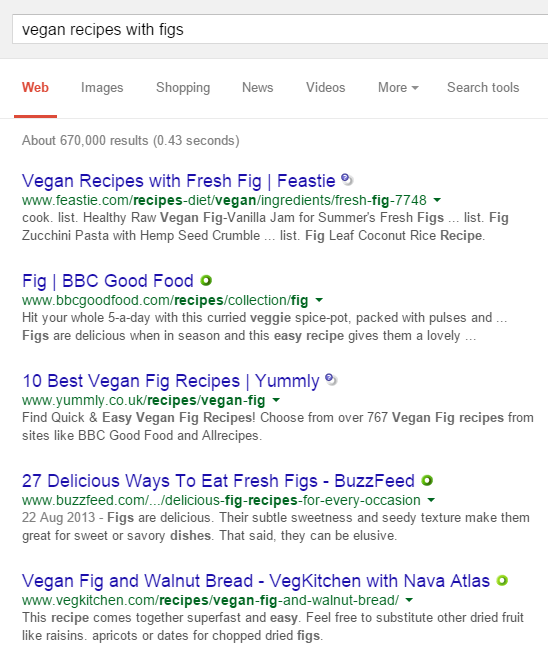The image depicts a Google search results page for the query "vegan recipes with figs." At the top, there is a search bar displaying the search query. Below the search bar, the web navigation section is highlighted in red, with a red underline, and includes options such as Web, Images, Shopping, News, Videos, More, and Search Tools, all in gray with a gray underline under this section.

The search results indicate there are about 670,000 results, fetched in 0.43 seconds. The first result is titled "Vegan Recipes with Fresh Figs" from Beasty, featuring dishes like raw vegan fig vanilla jam, zucchini pasta with hemp seed crumble, and coconut rice with figs. The second result is from BBC Good Food, with a recipe for a curried veggie spice pot that incorporates figs, ideal for a whole five-a-day serving. The third result lists "10 Best Vegan Fig Recipes" on Yummly, offering quick and easy options from various culinary websites including BBC Good Food and All Recipes. The final highlighted result is "27 Delicious Ways to Eat Fresh Figs" from Buzzfeed.